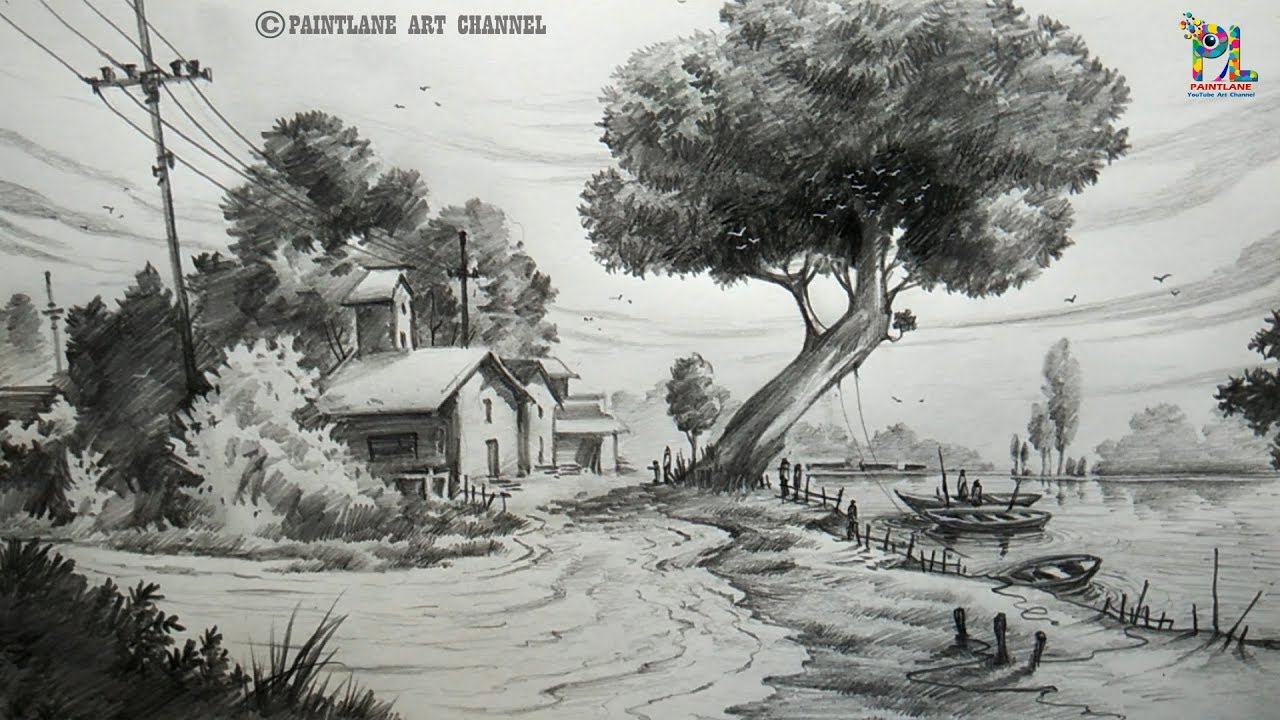This artwork, a black and white watercolor or pen and ink drawing, captures an idyllic country scene. The focal point is an older house, distinguishable by its chimney, situated near a lake. The house, partially surrounded by trees and shrubs, has a power line running behind it, and there's a dirt road leading up to it. A very large, rounded tree, growing from the front yard, extends high into the sky, which is rendered in swirling tones of gray and white clouds, giving the piece a somewhat dreary ambiance.

In the foreground, a swing hangs from the large tree, while a decrepit fence separates the land from the lake. The lake itself features three boats; one boat has small, discernible figures, though details are sparse due to their tiny size. Additionally, there are a couple of telephone poles with wires running along the dirt road, contributing to the rustic feel of the scene.

A copyright symbol appears in the upper left-hand corner, denoting the 'Paint Lane Art Channel,' and in the upper right-hand corner, the only color element is a small PL logo.细Additionally, the image features birds flying high, which are visible against the light-colored clouds, enhancing the overall earthy and serene atmosphere of this countryside depiction.